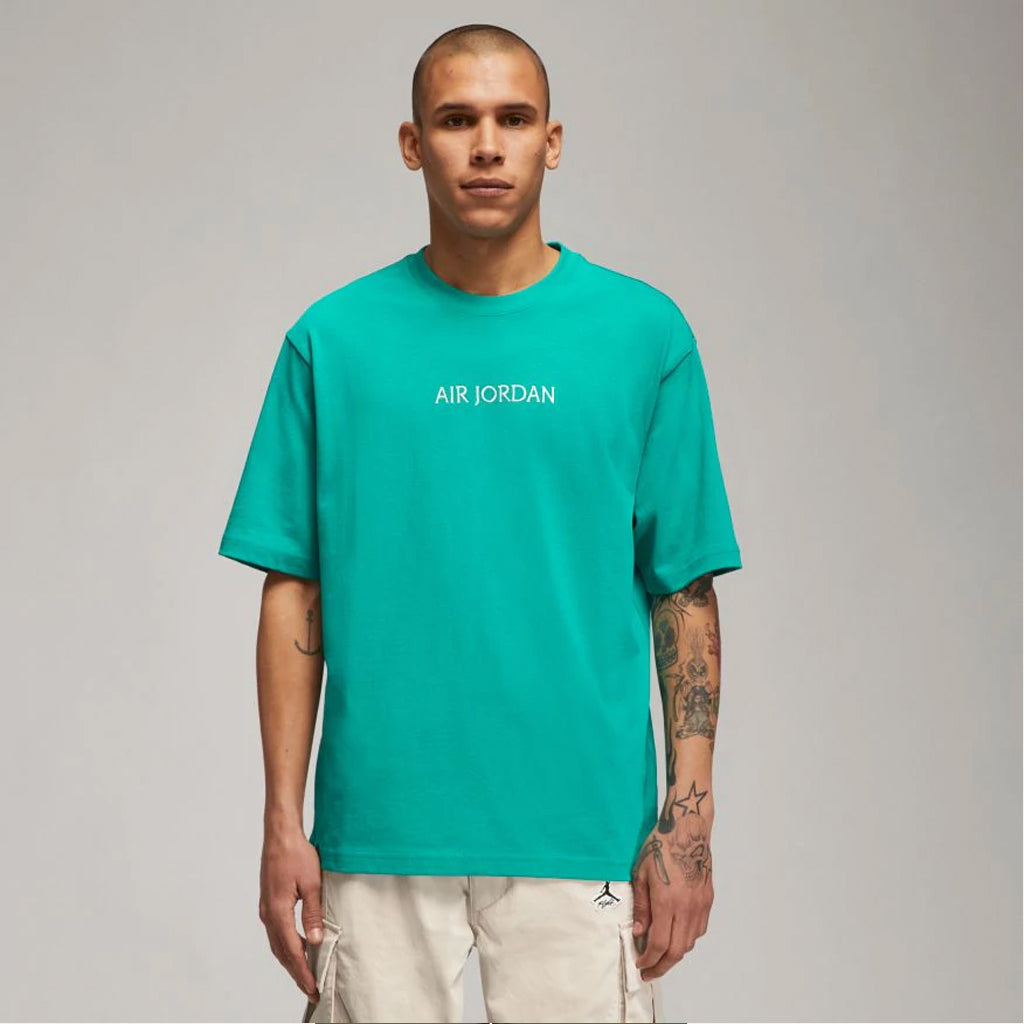The photograph features a young mulatto man in his early 20s, modeling a casual outfit against a light gray indoor background. The square image, approximately six inches by six inches, captures the model from mid-thigh up, standing in the center and facing the camera with a neutral expression. He has light brown skin, very short black hair with noticeable stubble, and distinctive facial features including dark eyes, a heavy brow, full lips, and wide ears.

He is wearing a loose-fitted, sea-green (teal) short-sleeved crewneck t-shirt with the words "Air Jordan" printed in small white letters across the chest. The shirt hangs untucked over tan (or white) cargo shorts, which feature a small black Air Jordan logo on the top of the right leg. Both of his arms are adorned with tattoos; the left arm is heavily tattooed with designs including a star, a tomahawk, skulls, an angry bunny rabbit, and a knife, while the right arm has a tattoo of a ship anchor near the inner corner of his elbow. His arms hang naturally by his sides, showcasing his tattoos prominently.